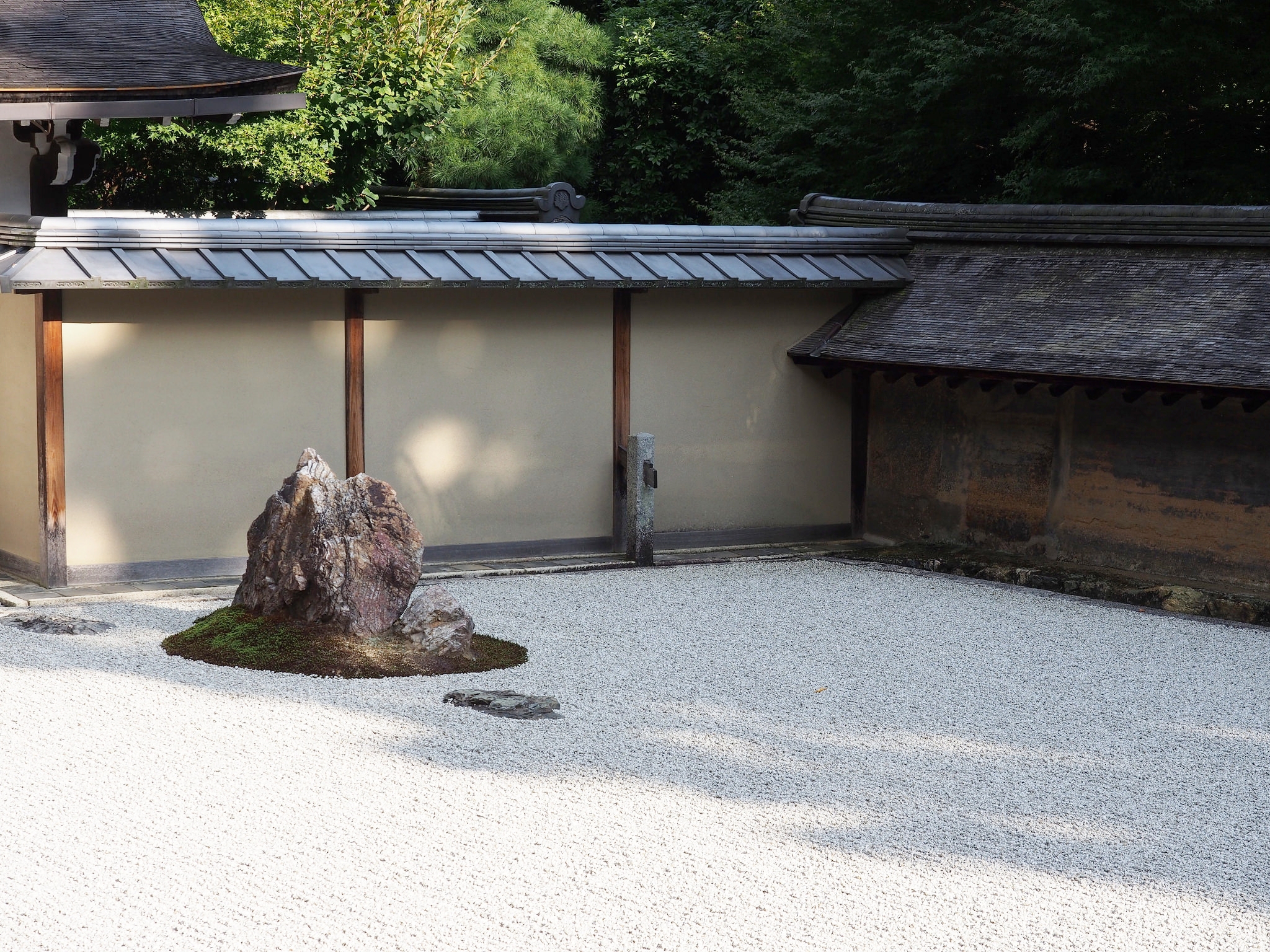The detailed image showcases a Japanese-style outdoor setting on a coarse, light gray to beige gravel ground. Dominating the center is an L-shaped structure formed by two single-level buildings of differing constructions. The left section, fashioned from large square light brown stones interspersed with wood beams, runs parallel to an older, more worn brown wooden building with a hipped roof on the right. The roofs of these structures appear to overlap slightly.

Amidst the gravel, slightly left of center, a stone feature stands about three feet tall. This notable centerpiece comprises a round platform topped with a large rock, resembling a miniature stone mountain or rock wall, positioned in front of a tan half-height wall divided by wood slats every few feet. 

In the background, verdant trees—one with light green leaves on the left and another with darker green leaves on the right—overhang the scenery, casting shadows over the ground and contributing to the ambiance. The trees' foliage is lush and vibrant, adding depth to the serene setting. Scattered throughout, areas of light and shadow interplay, suggesting the presence of sunlight filtering through the foliage. A rusted water pump lies off to the right, subtly blending into this tranquil garden tableau.